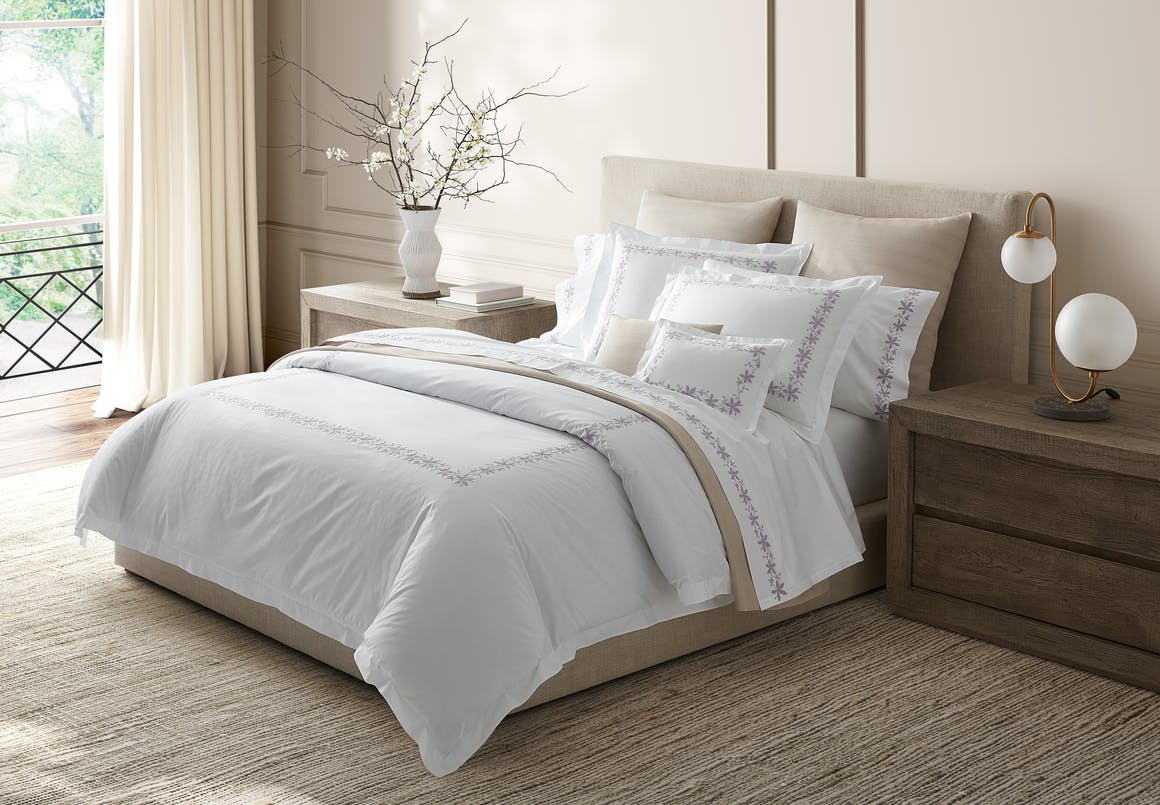The photograph captures an elegantly designed bedroom, reminiscent of a welcoming hotel room. The centerpiece is a queen-sized bed adorned with a plush white duvet cover accented by a delicate ridge of floral embroidery. A multitude of pillows, totaling seven, are meticulously arranged against the tan fabric headboard, including some in matching fabric and others in white with purple trim. On either side of the bed, there are matching nightstands; one features a gold lamp with dual white, circular lights of different sizes, while the other holds a vase with white flowers and several books. The window to the left offers a view of lush greenery and possibly a small deck or balcony, framed by large cream-colored curtains that are currently drawn open. The bed sits atop a flat, ridged rug placed over smooth hardwood flooring, completing the serene and inviting atmosphere of the room.